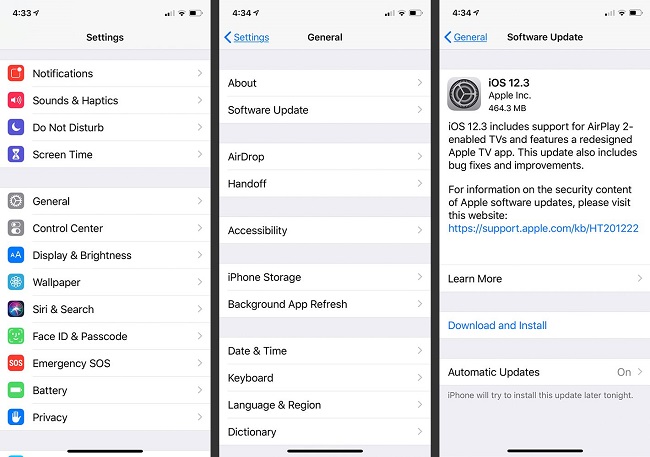The image showcases three clear and detailed screenshots of an iPhone’s settings interface. 

The first screenshot displays the main settings menu, enumerating various options such as "Notifications," "Sound & Haptics," "Do Not Disturb," "Screen Time," "General," "Control Center," "Display & Brightness," "Wallpaper," "Siri & Search," "Face ID & Passcode," "Emergency SOS," "Battery," and "Privacy."

The second screenshot drills down into the "General" settings category, listing sub-options like "About," "Software Update," "AirDrop," "Handoff," "Accessibility," "iPhone Storage," "Background App Refresh," "Date & Time," "Keyboard," "Language & Region," and "Dictionary."

The third screenshot examines the details of an "iOS 12.3" software update from Apple Inc., which is 464.3 MB in size. This update includes support for AirPlay 2-enabled TVs, features a redesigned Apple TV app, and incorporates various bug fixes and improvements for enhanced user experience.